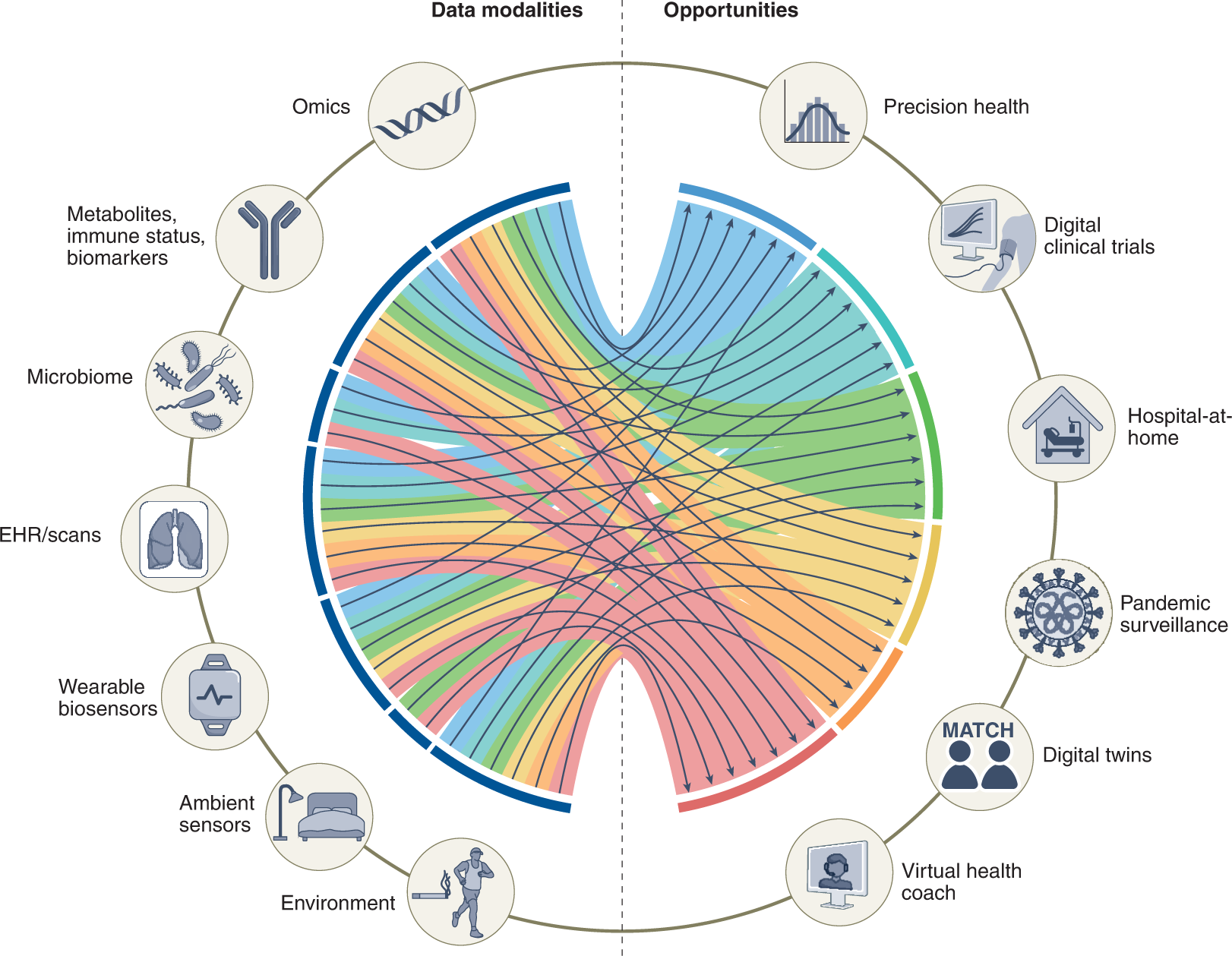Here's the concise, detailed caption:

---

The chart features a highly detailed infographic on a white background, resembling a science report. A central oval, horizontally divided by a blue dotted line, is bordered by arcs of varied colors on both left and right sides. The right side includes arcs of red, orange, yellow, green, and blue, while the left side is consistently blue. This oval has two notches on the top and bottom, forming a symmetrical design.

This diagram is framed by various icons in blue ovals, labeled with key concepts. On the right side from top to bottom, labeled "Opportunities," are icons for Precision Health, Digital Clinical Trials, Hospital at Home, Pandemic Surveillance, Digital Twins, and Virtual Health Coach. Conversely, the left side, titled "Data Modalities," features icons for Omics, Metabolites, Immune Status, Biomarkers, Microbiome, EHR Scans, Wearable Biosensors, Ambient Sensors, and Environment. Each icon is connected to the central oval by crisscrossing blue arrows, indicating their interrelations.

---